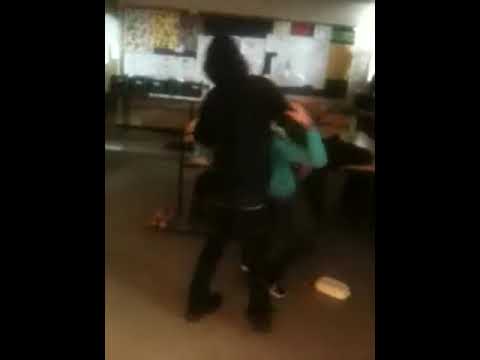This photograph, taken in what appears to be a school classroom, shows two figures standing with their backs to the camera. The larger individual, potentially an adult, is dressed entirely in black, wearing a hooded sweatshirt, jeans, and sneakers, with the hood pulled up. This person has their right arm around a smaller figure or child, who is wearing a teal long-sleeve shirt, dark pants, and dark shoes. The child's face is not visible. The scene, slightly blurred, suggests a moment of rough play or a potential altercation, as the larger person appears to be gripping the smaller one around the neck.

The classroom setting is marked by a beige or light gray hard surface floor and features several tables scattered with various items. A white square object is seen on the floor to the right. Vertical black bars frame the sides of the image, further emphasizing the central action. In the background, there is a wall adorned with posters and colored signs, characteristic of a school environment. Light filters dimly through windows on both the left and right, adding a subtle illumination to the otherwise unclear image.